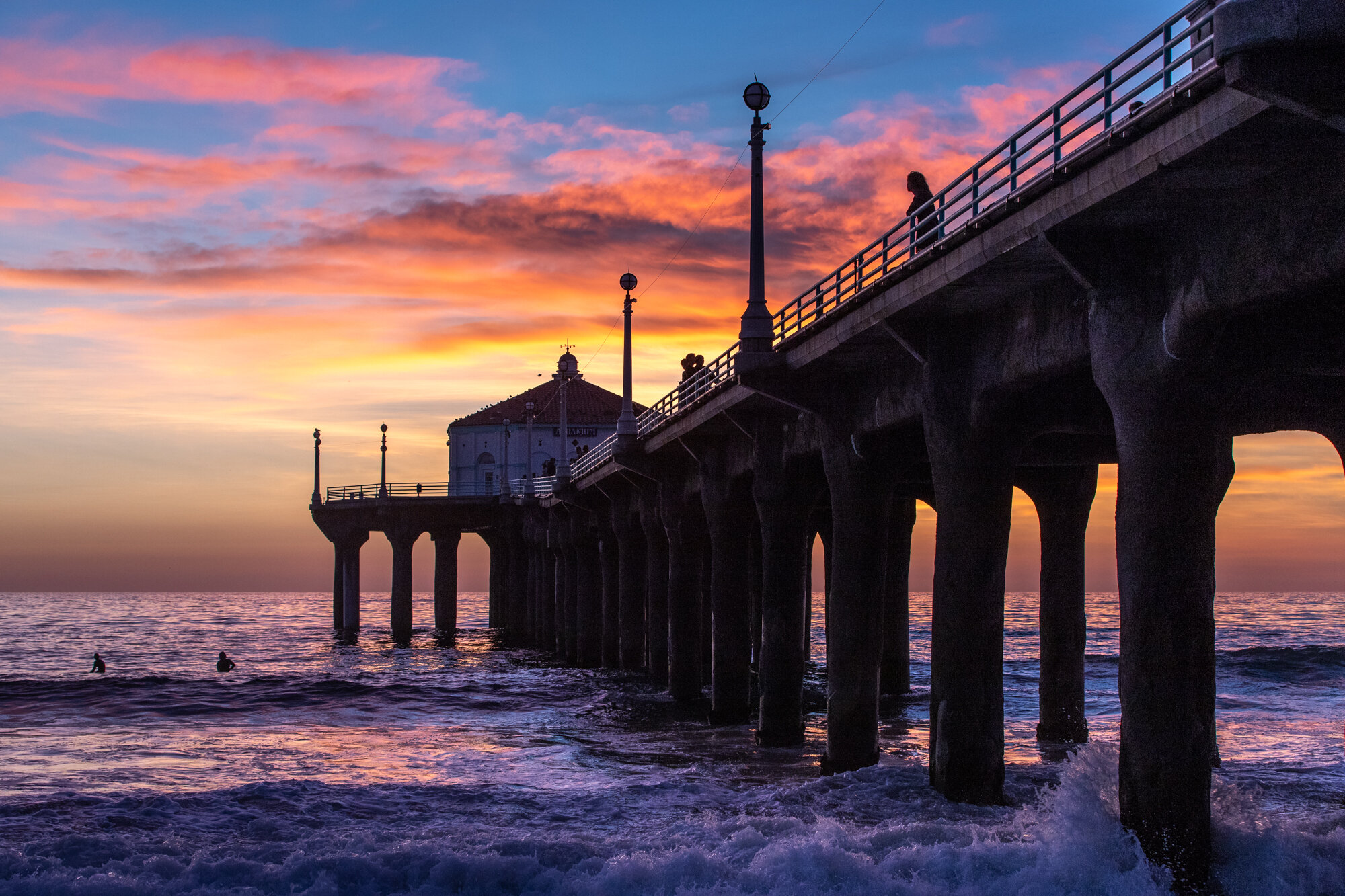The photograph captures a serene sunset scene over an ocean, with the sky transitioning from dark blue at the top to vibrant hues of orange, yellow, and pink near the horizon. The centerpiece of the image is a tall boardwalk, supported by numerous towering concrete pillars that rise above the water. Waves gently splash against these massive legs. The boardwalk, also made of concrete, features a metal barrier along its edge and is dotted with lamp posts crowned by small orbs, likely the lamps themselves. A small white building with a terracotta, pointed roof, and a cross at its peak stands at the end of the boardwalk, adding a quaint charm. The water below reflects the sky's stunning colors, appearing as a mix of dark indigo and purple. Two figures can be seen in the water near the bottom left, while another person stands at the edge of the boardwalk, gazing out at the tranquil scene. Above, a few birds rest on the water, completing this picturesque sunset view.